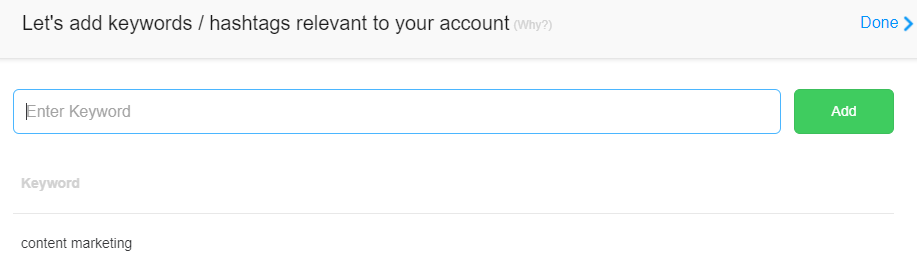The top portion of the image features a light gray rectangle stretching across its entirety. Within this rectangle, black text reads "Let's add keywords / Hashtags relevant to your account." Approximately five inches to the right, the word "Done" is displayed in blue, accompanied by a small right-facing arrow.

Below this, there is a text box outlined in blue containing a vertical line with gray placeholder text that says "Enter keyword." To the right of this text box, within a green rectangle roughly three inches in length, the word "Add" appears in white text.

Further down, about two inches to the left, the word "Keyword" is displayed in light gray. Below this, another two inches down, in a smaller font, are the words "Content Marketing," both in black text.